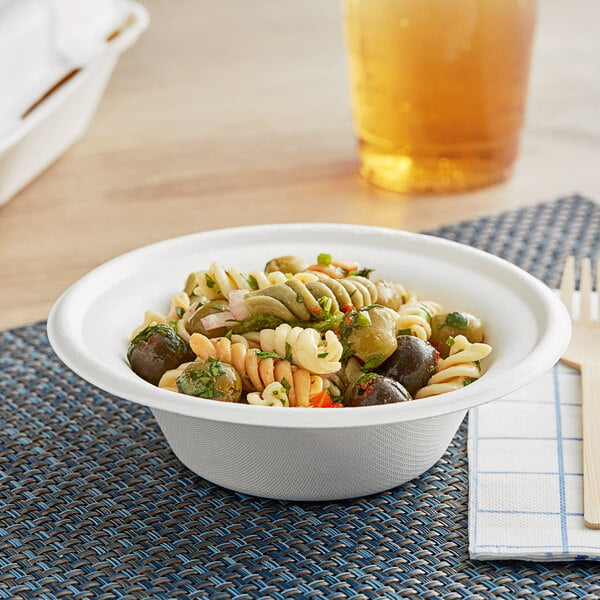In this beautifully composed photograph reminiscent of a food magazine, we observe a delicious pasta salad presented in a plain white bowl, centrally positioned on a wooden table. The vibrant pasta, featuring colorful spirals of green, yellow, and orange, is complemented by olives and garnished with a green leafy herb. The appetizing meal is set against a bluish-gray woven placemat, adding texture to the scene. To the right of the bowl, a white napkin adorned with a thin blue checkered pattern holds a wooden fork, enhancing the table's rustic charm. A glass of what appears to be a yellow-orange beverage, possibly tea or apple juice, sits at the top right corner, while the top left reveals a partially visible white takeout box, suggesting a cozy, ready-to-enjoy meal. The entire setting captures a moment of anticipation, inviting the viewer to imagine the flavors and enjoyment to come.